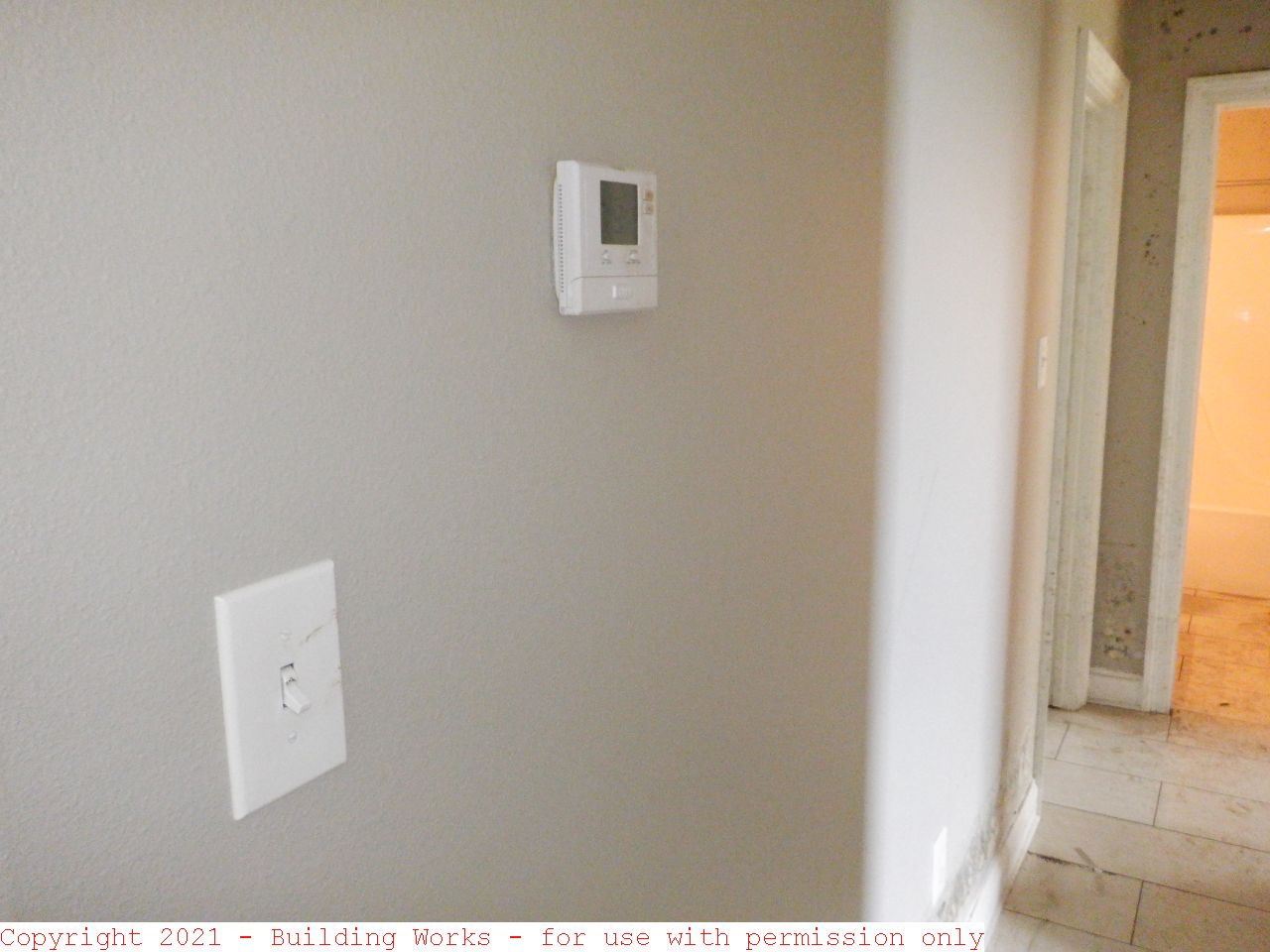This photograph showcases the interior of a dilapidated, empty house. Taken in 2021, the image is marked with "Copyright 2021 Building Works For Use With Permission Only" at the bottom. The primary focus is a gray wall, marred by severe damage, situated at the front. On the left section of this wall, a white light switch and a digital white thermostat are noticeable. The degradation continues down the wall, characterized by bubbled and peeling paint, suggestive of potential water damage. The tile floor below is equally distressed, with visible separation and a layer of dirt covering its surface. There is no furniture visible, emphasizing the desolation of the space. Additionally, a worrying presence of what appears to be black mold is observed at the bottom of the wall. Two doorways branch out from this area, one leading left and the other right, hinting at further rooms likely in a similar state of disrepair.